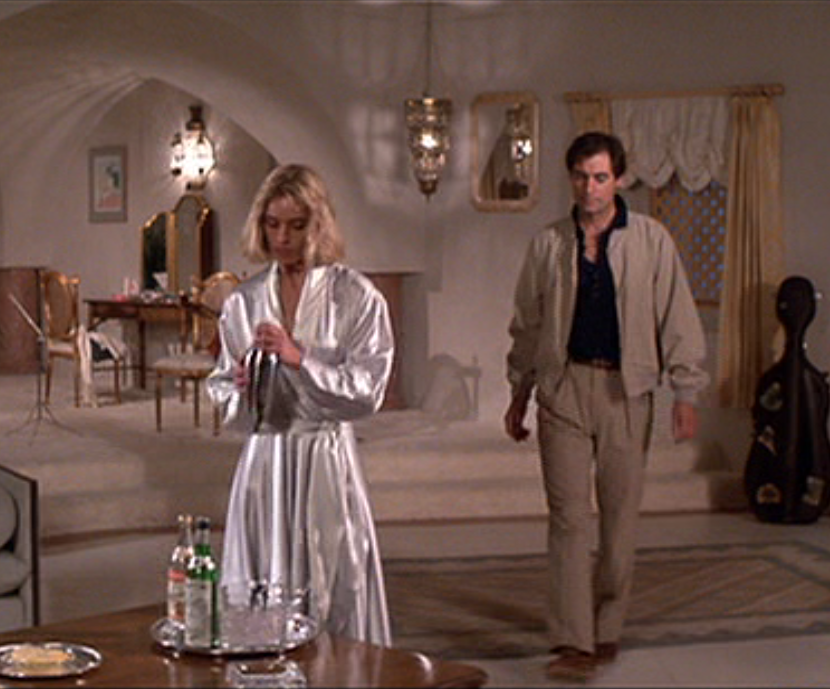The image appears to be a still from a movie or TV show, set within a luxurious, monochromatic apartment. The scene is defined by beige flooring, beige walls, and a tan carpet. In the lower left corner, there is a tan dining table with a tray holding an ice bucket and two bottles of liquor, accompanied by a chair slightly pulled out. Farther in the background on the left, up three steps, is a dark brown dining table with two chairs pulled out and a light fixture suspended overhead. Centered in the image hangs another light fixture, while a window with brown drapes and a tan awning is visible on the right side, near a dark cello case.

In the foreground, a man dressed in beige pants, a beige jacket, and a black shirt is walking towards a woman. The woman, wearing a white silk robe, stands behind the liquor table, concentrating on a silver drink mixer in her hands. She appears to be making a cocktail. The opulent room and the formal attire of the individuals suggest a scene rich in tension and elegance, possibly from a classic film, as the image quality hints at an older cinematic style.